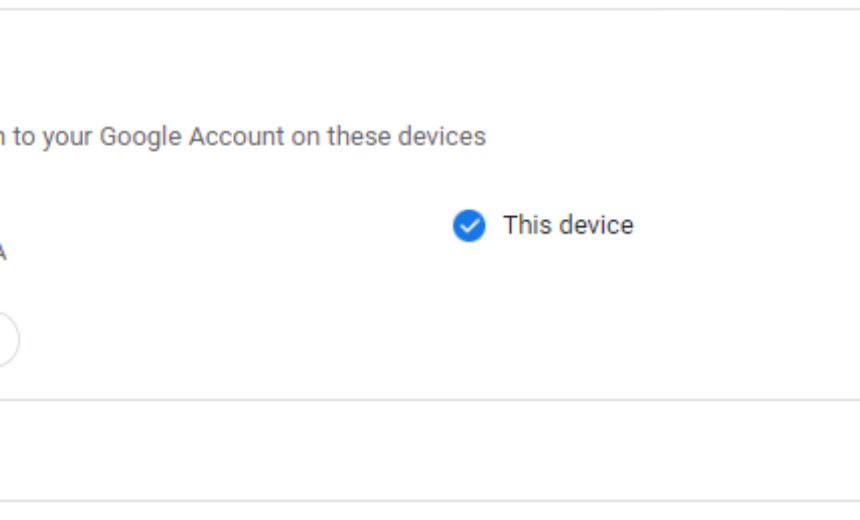The image features a white background with a graphical representation of a half-circle and the bottom portion of a cursor or arrow. In the middle of the half-circle, there are two parallel horizontal lines with a segment of text between them, providing information related to a Google account. Below this section, there's a third horizontal line. Additionally, within the composition, there's a blue circle containing a white checkmark, accompanied by the phrase "this device."